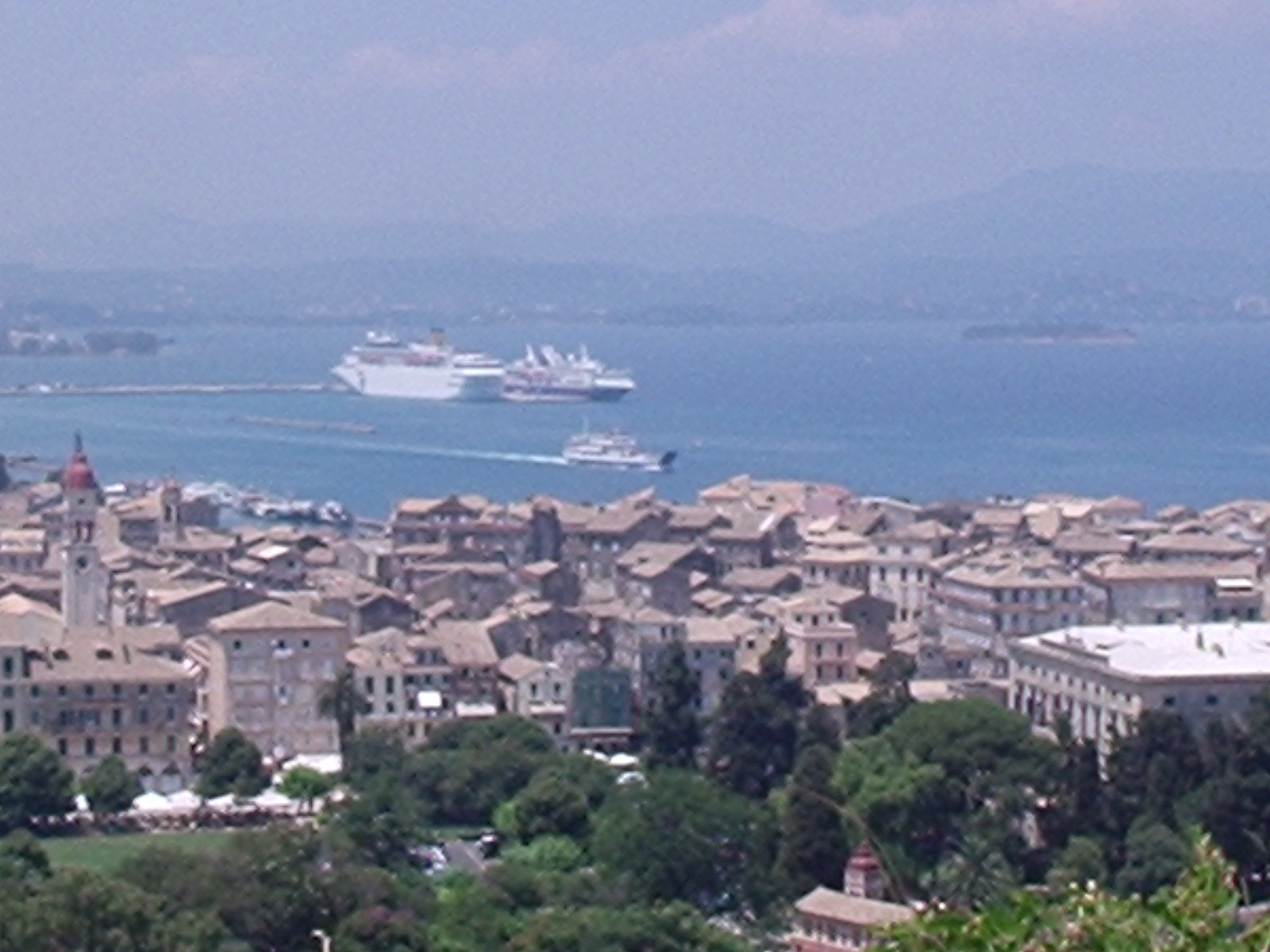This photo, taken from a high vantage point, captures a cityscape overlooking a harbor against a backdrop of distant mountains. The foreground features a neatly cared-for lawn and a series of trees, with one notable building nestled among them. The city itself is composed of predominantly brown and white buildings, displaying a European architectural style. In the very foreground is a larger, possibly government building. The harbor, situated in the middle of the image, shows clear blue water with various ships, including two large cruise ships and a smaller one nearby. The ships sail outward from a dock area on the left, leaving visible white wakes behind them. The top half of the photo reveals a hazy, mountainous horizon under a gray sky, suggesting it might be an older or low-resolution image. The scene is serene, depicting a clean, orderly, and pleasant city by the sea.